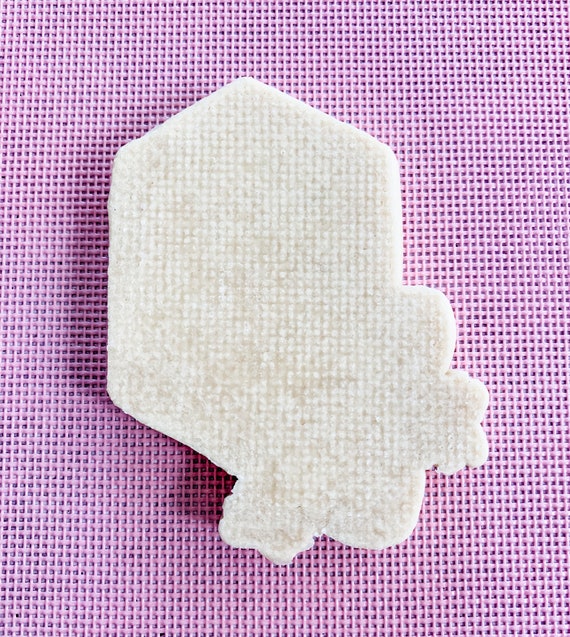A minimalist image showcasing a white object, which resembles a house with a cloud-like shape on its lower right side, resting atop a textured, deep purple mat. The mat displays a tightly knit, square pattern reminiscent of kitchen materials, with a matte finish that adds a subtle, aesthetically pleasing touch to the overall composition.